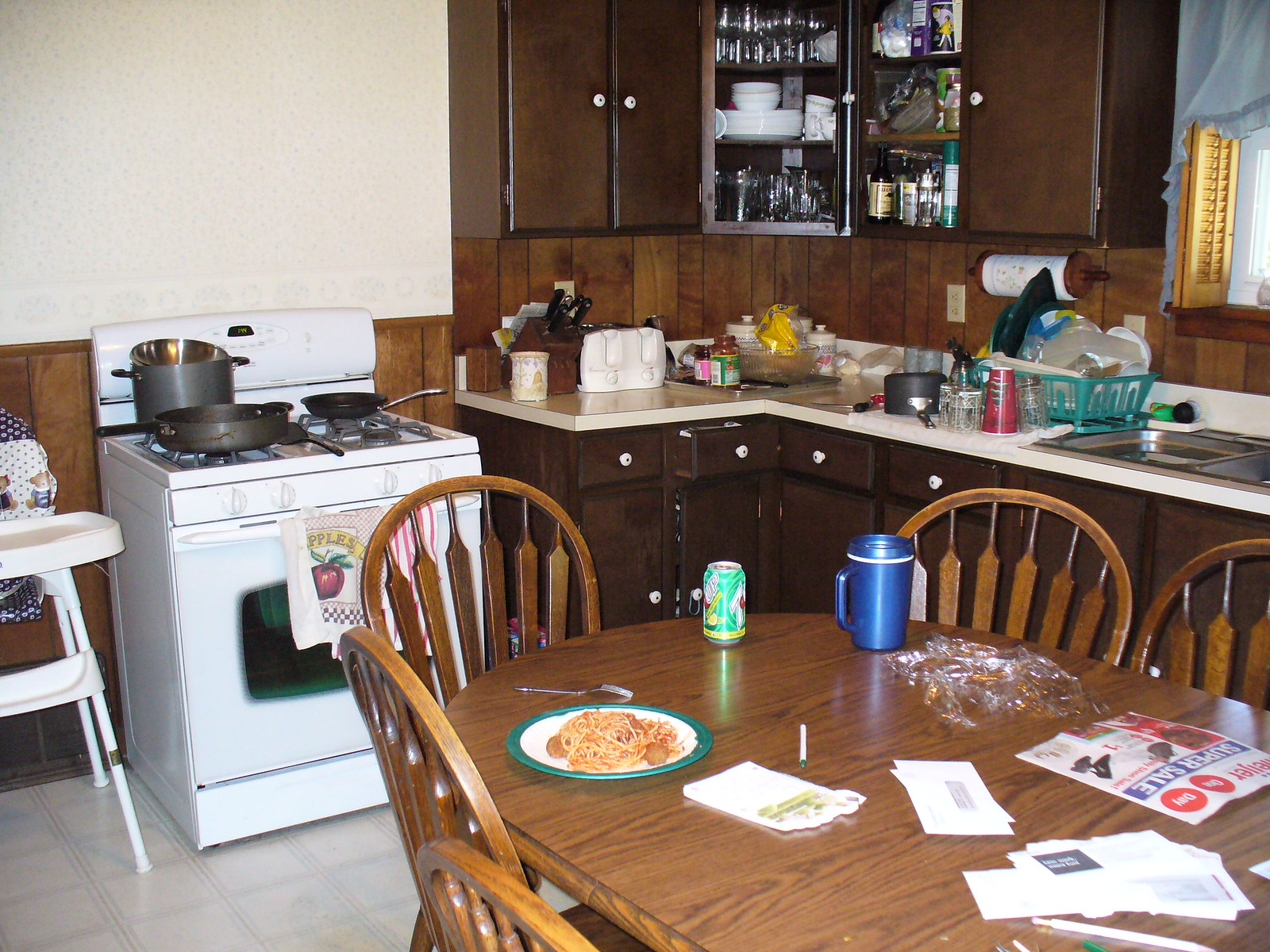The image captures a cozy, well-used kitchen filled with various elements of daily life. The top half of the room features a pristine white wall, while the lower half is adorned with white wood paneling. In the bottom left corner, a kiddie chair with long legs and a small tray is placed, designed to safely seat toddlers during mealtime.

An oven stands prominently in the background with a towel hanging on it. Above the stove, a pan sits to the left and pots occupy the back right burner. In front of the stove, a wooden table is laden with various items. The table is surrounded by wooden chairs with intricate line designs and arching backs.

On the left side of the table, a plate brimming with spaghetti and meatballs sits invitingly. To the right, scattered mail shares space with a blue cup. In the back of the room, a countertop hosts multiple kitchen appliances and items, including overturned cups, a drying rack filled with plastic containers, and a roll of patterned paper towels.

Above the countertop, an open cabinet reveals a collection of glasses, bowls, dishes, and bottles, along with a blue cylindrical salt container bearing an iconic image of a little girl in a yellow raincoat holding an umbrella. An open window to the right is framed with wood paneling, blinds, and a delicate curtain at the top, allowing a glimpse of the outside world.